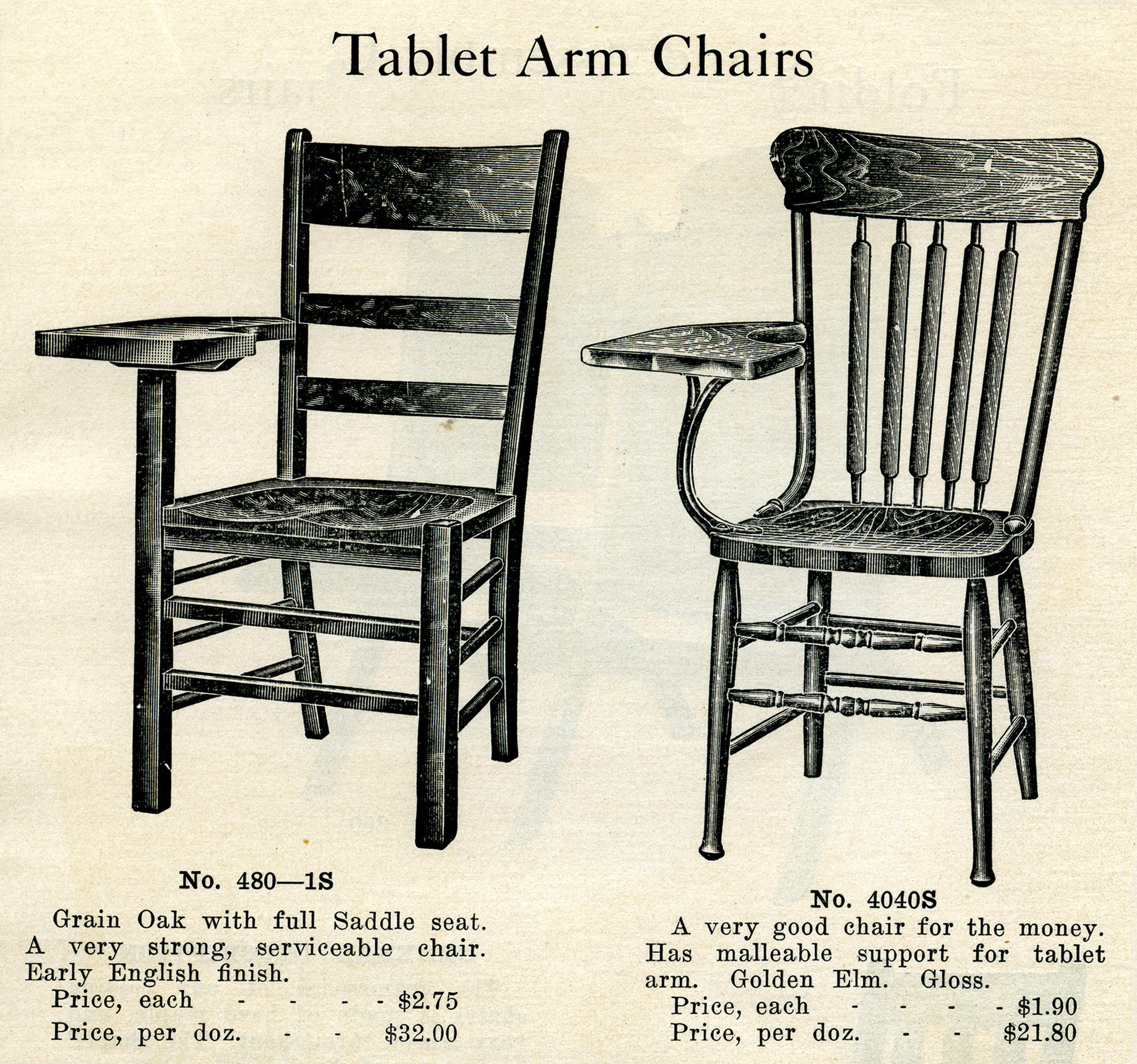The image is an antique advertisement for two types of tablet armchairs, depicted in black and white illustrations on a light beige background. At the top, the title "Tablet Armchairs" is prominently displayed in black text. The first chair on the left, identified as number 480-1S, is crafted from grain oak with a full saddle seat and an early English finish. This chair, described as very strong and serviceable, features a backrest with two horizontal slats and one thicker horizontal piece at the top. It is priced at $2.75 each, or $32 per dozen.

The second chair, on the right, labeled as number 4040-S, is described as a very good chair for the money. It has a rounded backrest with five vertical slats and a malleable support for the tablet arm, finished in a golden elm gloss. Its price is $1.90 each, or $21.80 per dozen. Despite the grayscale presentation, the intricate carvings and sturdy design details of both chairs are clearly visible, highlighting their quality and durability.